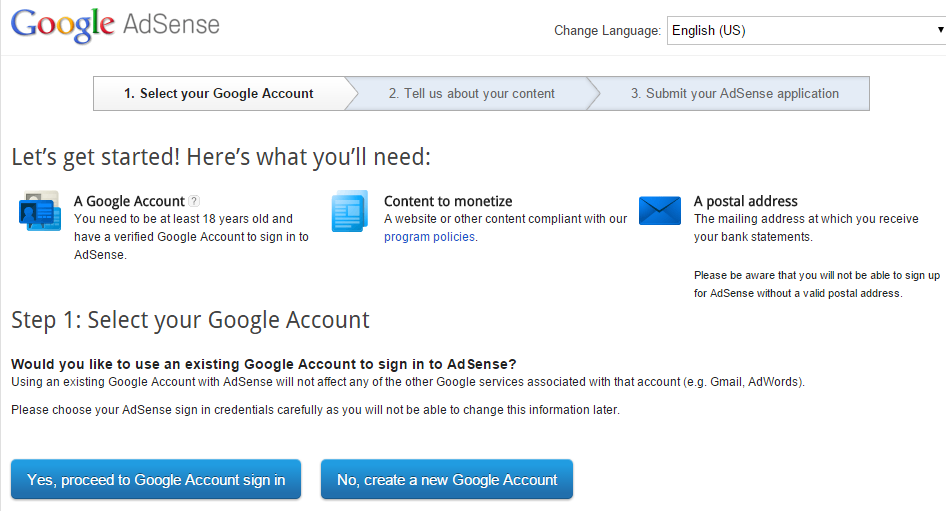The screenshot displays a step-by-step guide for setting up a Google AdSense account. 

At the top, there's a header labeled "Google AdSense" and an option to change the language to English (US). The step-by-step instructions are as follows:

1. **Select your Google account:** Choose an existing Google account to sign in to AdSense. Using an existing account will not affect your access to other Google services (e.g., Gmail, AdWords). It's important to select your AdSense sign-in credential carefully since it cannot be changed later.

2. **Tell us about your content:** Provide details about your website or other content that you wish to monetize. Ensure that it complies with AdSense program policies.

3. **Submit your AdSense application:** Complete the application process by providing a valid postal address where you receive your bank statements. Note that you must be at least 18 years old and have a verified Google account to sign up.

A prompt at the bottom reads, "Let's get started," outlining the main requirements: a verified Google account, content to monetize, and a postal address.